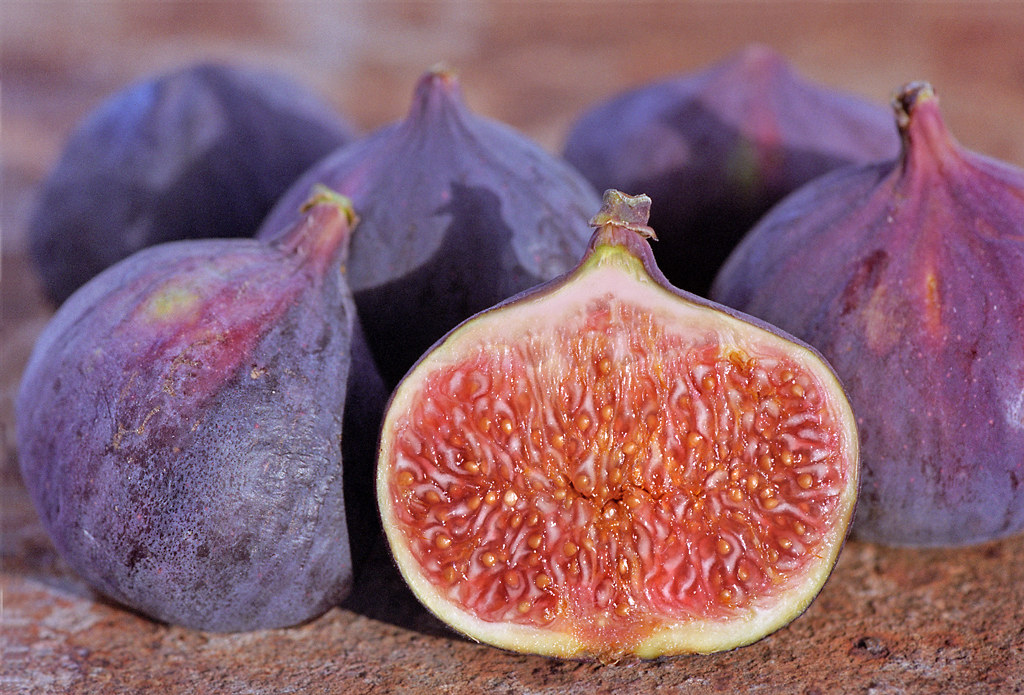This vibrant color photograph, captured in landscape orientation, showcases an intimate macro view of six figs arranged in two rows, with two figs in the back, two in the middle, and two in the front. The figs, displaying a deep purple hue with tinges of yellow and lighter pinks, have a rustic charm as they lie atop a rough, reddish-brown textured surface that resembles rocky dirt.

In the forefront, the rightmost fig is sliced open, revealing a stunning cross-section. The perfectly halved fig exposes its juicy, vibrant interior: a crisp white outline framing a rich, reddish flesh packed densely with dark red seeds, some tinged with shades of orange and brown. The seeds are surrounded by a glossy, jelly-like substance, while delicate white fibers weave through the flesh, enhancing the fig's fresh and succulent appearance. The well-lit composition emphasizes the intricate details and textures of the figs, making them appear freshly cut and invitingly juicy. In the blurred background, a mix of brown and white tones adds depth, directing the focus to the figs and their striking interior.